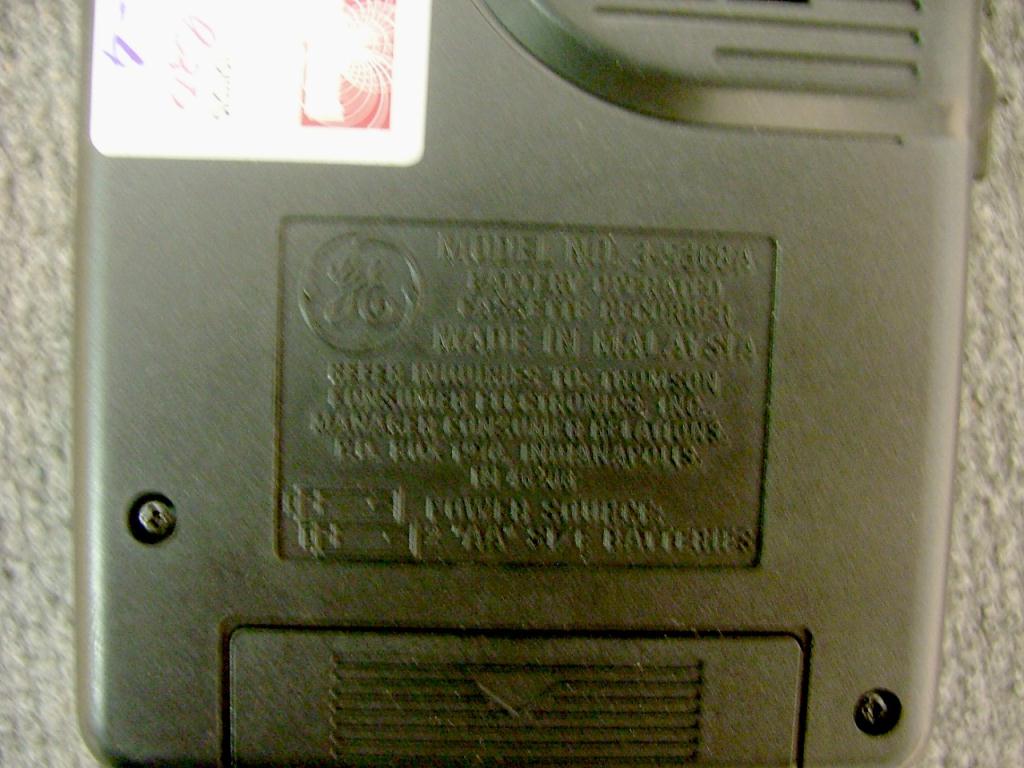This photo captures what appears to be the bottom portion of a gray, metallic electronic device, possibly a fuse box or a doorbell, mounted on a gray and white textured wall. The device is square-shaped, taking up nearly the entire frame of the photo. Prominently displayed in the center is the embossed GE (General Electric) logo inside a circle, although the details surrounding the model number and other specifications are too blurry to read. The label does indicate it was made in Malaysia. Below the logo, there is a small drawer-like area, potentially a battery compartment, indicated by an arrow pointing downwards. The compartment appears to be around four to five inches long. Additionally, there are two visible screws: one in the bottom right corner and another on the left side, just above the battery access door. Affixed to the top left corner is a bright white label with a red and white pattern, possibly suggesting its use as a doorbell with a push-button feature.